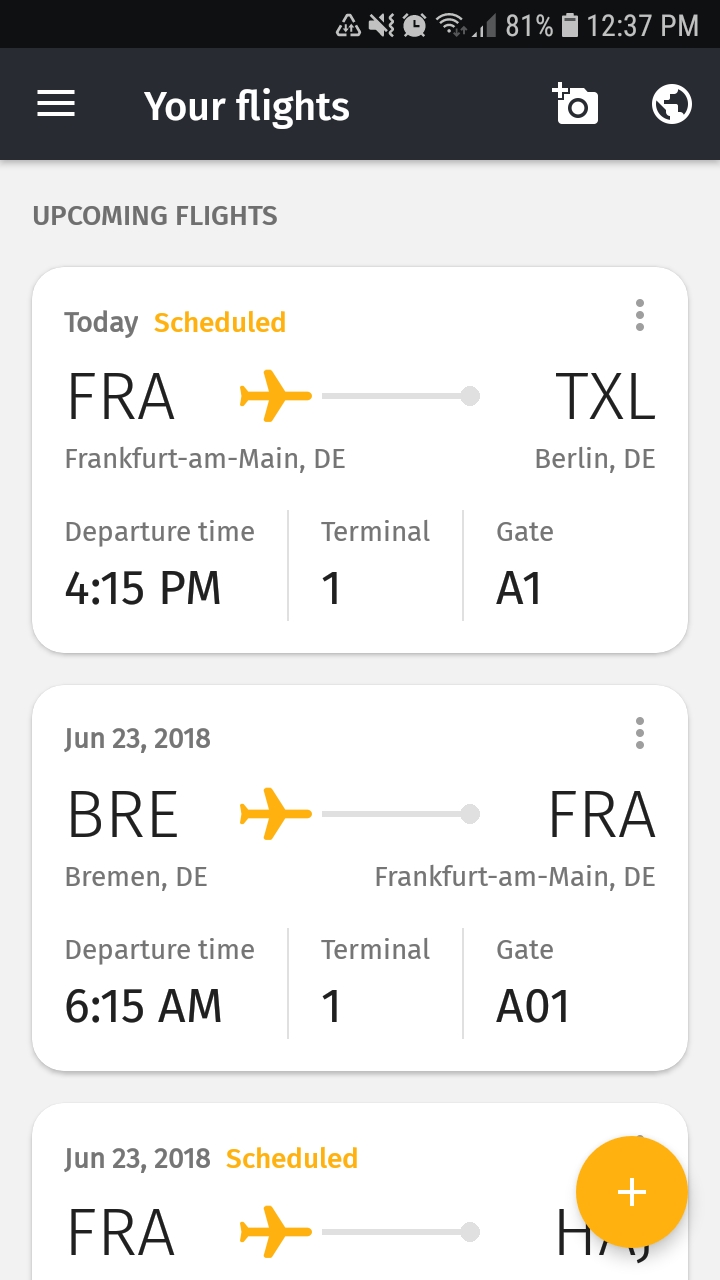The image depicts an individual reviewing their flight options, likely from an online airline portal. While the specific airline is not identifiable, the details of various flights are clearly visible.

At the very top right corner of the screen, a number of system indicators are displayed: upload and download icons, no alarm, sound disabled, an active alarm set, full Wi-Fi connectivity, half-signal bars, battery at 81%, and the current time reading 12:37 PM. Below these indicators, there is a hamburger menu on the left. In large, white text in the center is "Your Flights," accompanied by an "Add a Photo" button and a world icon on the right.

In the white area beneath this header, a section labeled "Upcoming Flights" is visible. This section features rectangular panels with rounded corners and subtle drop shadows to enhance readability.

The first panel indicates a flight scheduled for today. It uses a yellow plane icon with a dot and a bar to designate the start and end points. The flight is from Frankfurt (FRA) to Berlin (TXL) in Germany, departing at 4:15 PM from Terminal 1, Gate A1.

The second panel details a flight from Bremen (BRE) to Frankfurt (FRA) on June 23, 2018, at 6:00 AM, departing from Terminal 1, Gate A01.

The third panel shows a flight from Frankfurt (FRA) to Hannover (HAJ). However, a yellow circle with a plus sign overlays the destination, partially obscuring the details. Additionally, the departure time, terminal, and gate information are cut off at the bottom of the panel. 

Overall, the image provides a comprehensive view of the person's upcoming travel itinerary, complete with specific flight details and navigational elements.